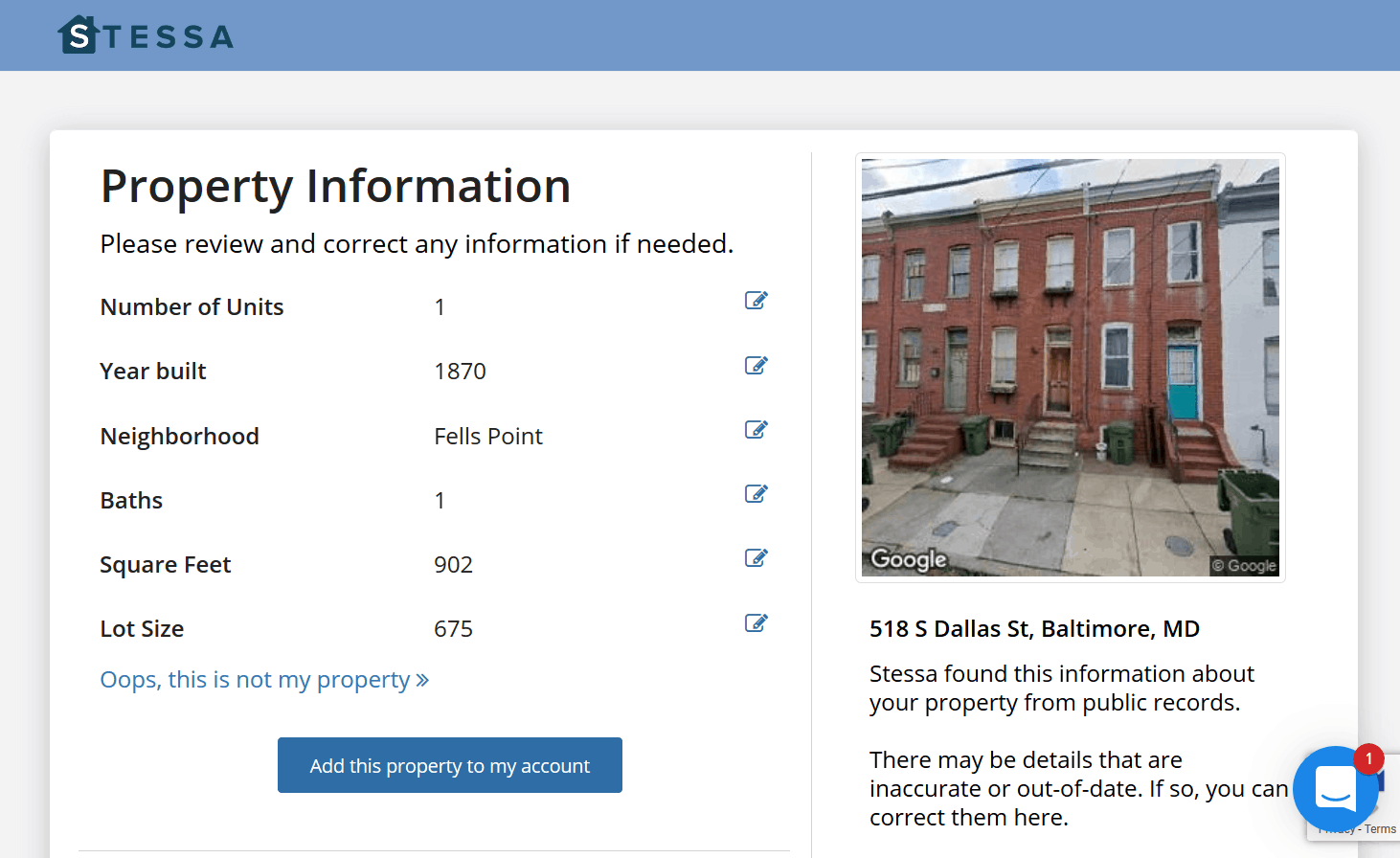The top left corner of the image features text with "S" enclosed in a house-shaped design in white, and "Tessa" outside the house, written in dark blue against a blue background. Below this, the background turns white, where text on the left reads, "Property Information. Please review and correct any information if needed." Each section has a blue date button on the right side. The first section lists "Number of Units: 1," "Year Built: 1870," "Neighborhood: Fence Point," "Bath: 1," "Square Feet: 902," and "Lot Size: 675."

At the bottom, a text reads, "Oops, this is not my property," in blue with the preceding text in black. Below it, there's a blue button with white text stating, "Add this property to my account."

On the right side, an image showcases a brick building with some green trash cans in front. The address, "518 Estella Street, Baltimore MD," is displayed. Additionally, a text notes, "Tessa found this information about your property from public records. There may be details that are inaccurate or out of date. If so, you can correct them here."

Finally, on the bottom right, there's a blue circle with a white conversation icon, alongside a red circle featuring a contact us conversation icon.